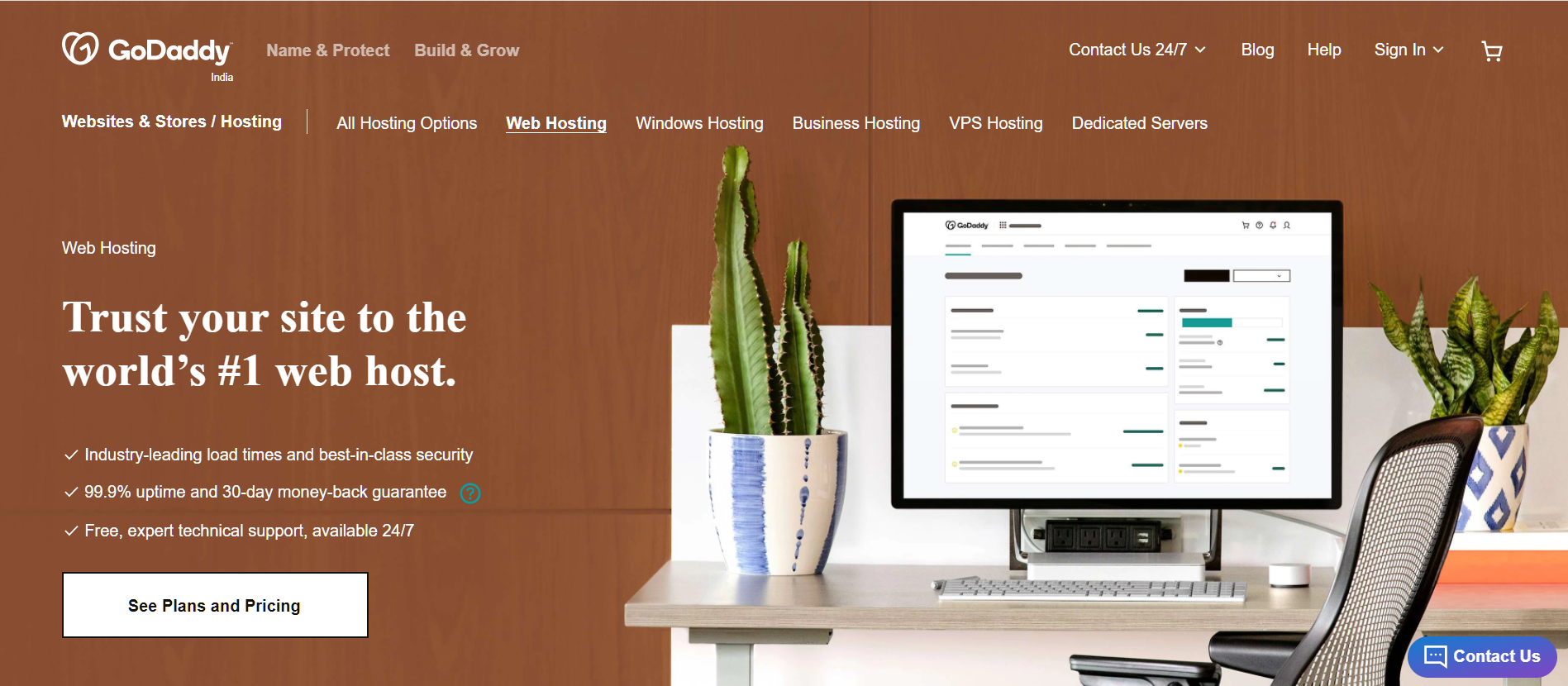The image depicts a GoDaddy website, featuring an interface with a detailed layout showcasing various hosting options. The website background mimics wood paneling, resembling a decorative wall. A wooden desk, possibly made of light ash wood, supports a computer monitor. On the desk, to the left of the monitor, sits a white-potted cactus, and to the right, a small spider plant in a blue pot. The ergonomic office chair in front of the desk has a webbed design.

In the upper left corner of the website, the text "GoDaddy India" is prominently displayed. Nearby, text emphasizes key services: "Protect, Build, and Grow." The upper right section offers navigation options including "Contact Us 24/7," along with dropdown menus for "Blog," "Help," "Sign In," and a shopping cart icon.

The next line of navigation options includes:
- Websites & Stores / Hosting
- All Hosting Options
- Web Hosting (highlighted)
- Windows Hosting
- Business Hosting
- VPS Hosting
- Dedicated Servers

On the left side, a section labeled "Web Hosting" offers the following features:
- "Trust your site to the world's number one web host"
- "Industry-leading load times"
- "Best-in-class security"
- "99.9% uptime"
- "30-day money-back guarantee"
A small green question mark in a circle icon appears nearby for additional information.

Below these details, the website advertises "Free expert technical support available 24/7," with a prominent button inviting users to "See Plans and Pricing."